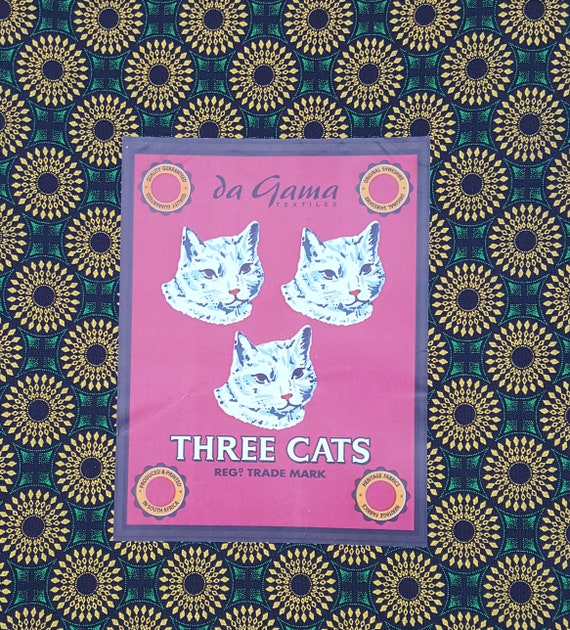This image is a vibrant, retro-style print, likely the cover of a product by Degama Textiles showcasing their "Three Cats" pattern. The design features a dynamic kaleidoscope background in hues of blue and yellow with convex squares and yellow mandalas interspersed. At its heart, a dark pink rectangular card is bordered by a dark gray color and prominently displays the text "Degama Textiles" and "Three Cats, registered trademark." The centerpiece of the card showcases three beautifully shaded white cats with bluish and dark accents and pink noses, with two cats arranged at the top and one at the bottom, all perfectly centered. The card also contains four corner circles with pink interiors set against a dark teal and light gold background featuring numerous gold circles outlined with dark teal. The overall aesthetic is completed with fine detailing, highlighting its quality and origin as produced and printed in South Africa.